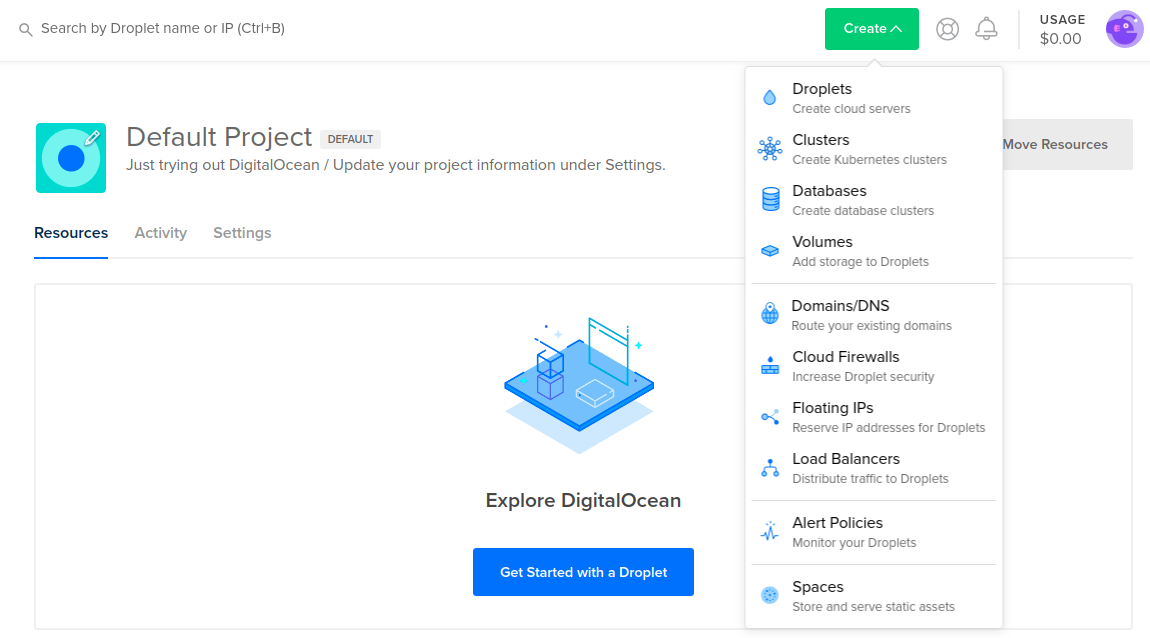The image depicts a DigitalOcean user interface with a clean, white background. At the top, there is a small, gray shaded search bar displaying the prompt "Search by droplet name or IP" with a shortcut hint "CTRL + B" in parentheses. To the left of the search bar, a gray banner reads "Default Project," with "default" in black.

Below this section, a green square contains a turquoise circle with a blue circle in the center, marked by a white pencil icon at the bottom right corner. Adjacent text states, "Just trying out DigitalOcean / update your project information under settings."

Menu options are displayed horizontally with "Resources" highlighted in black with a blue underline, while "Activity" and "Settings" appear in gray. Two fine gray lines visually separate these sections.

In the middle-right area of the interface, a blue diagram is showcased. Beneath it, text in black reads "Explore DigitalOcean." A prominent blue banner below this invites users to "Get started with a droplet" in white letters.

On the right side, a vertical navigation banner lists various cloud services. Each service is accompanied by a blue icon and a description:

- "Droplets" shows a blue droplet and states "Create cloud services."
- "Clusters" features a blue cluster icon with "Create Kubernetes clusters."
- "Databases" displays stacked blue coins with "Create database clusters."
- "Volumes" shows a blue box indicating "Add storage to droplets."
- "Domain DNS" has a blue circle with a teardrop icon, reading "Route your existing domains."
- "Cloud firewalls" demonstrates a blue box with a dot, saying "Increase droplet security."
- "Floating IPs" accompanied by an unidentified blue icon mentions "Reserve IP addresses for droplets."
- "Load Balancers" includes an icon resembling headphones with "Distribute traffic to droplets."
- "Alert Policies" features a blue graph icon, stating "Monitor your droplets."
- "Spaces" shows a blue circle with "Store and serve static assets."

Above this box, a green banner with white text reads "Create," alongside a gray bell icon indicating notifications. Additionally, there is a section showing "Usage: $0," marked by a purple circle with a small purple alien icon. Lastly, text on the white background reads "Move resources."